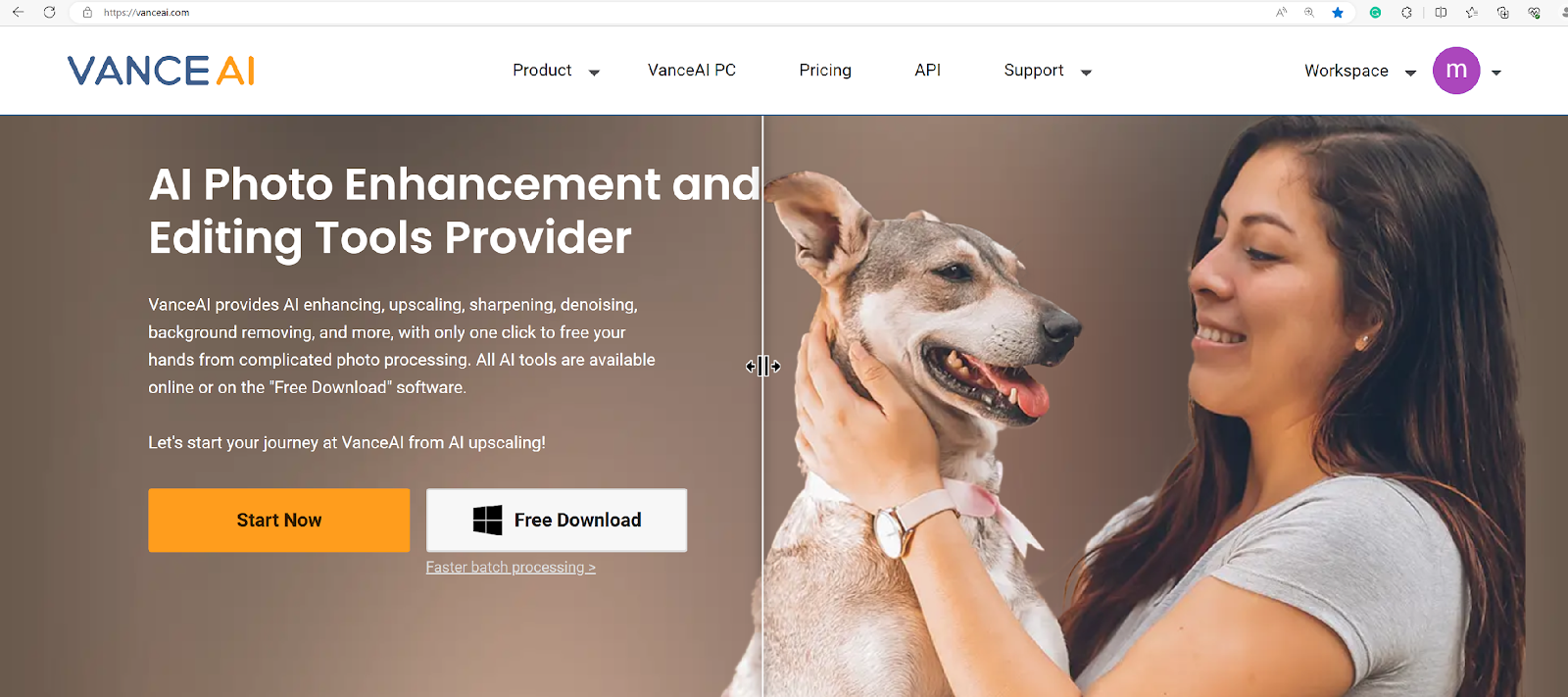The screenshot showcases the homepage of the Vance AI website. At the top, there is a navigation bar with a white background featuring the "Vance AI" logo, where "Vance" is in blue and "AI" is in orange. Above this, there is a browser tab with a search bar displaying "vanceai.com," along with refresh and back arrow buttons. On the right side of the tab are the usual browser buttons for favorites and settings.

Directly to the right of the "Vance AI" logo, there is a series of menu items: "Product" with a drop-down menu, "Vance AI PC," "Pricing," "API," and "Support" with another drop-down menu. Further to the right, there is a "Workspace" drop-down menu and a logged-in section indicated by a purple profile icon with the letter "M."

Below the navigation bar is a main banner image featuring a young woman with long brown hair, wearing a gray shirt and a pink watch. She is joyfully holding a brown and white two-tone dog with a black nose. The background of the banner is brown.

Overlaid on the image is a text description in white, promoting Vance AI as a provider of AI photo enhancement and editing tools. The text highlights the platform's capabilities, including AI-enhancing, upscaling, sharpening, denoising, and background removal, all available with one click. It mentions that the AI tools are accessible online or via free downloadable software. The call to action encourages users to start their journey with Vance AI, specifically with AI upscaling, and provides a "Start now" prompt along with a "Free Download" button.